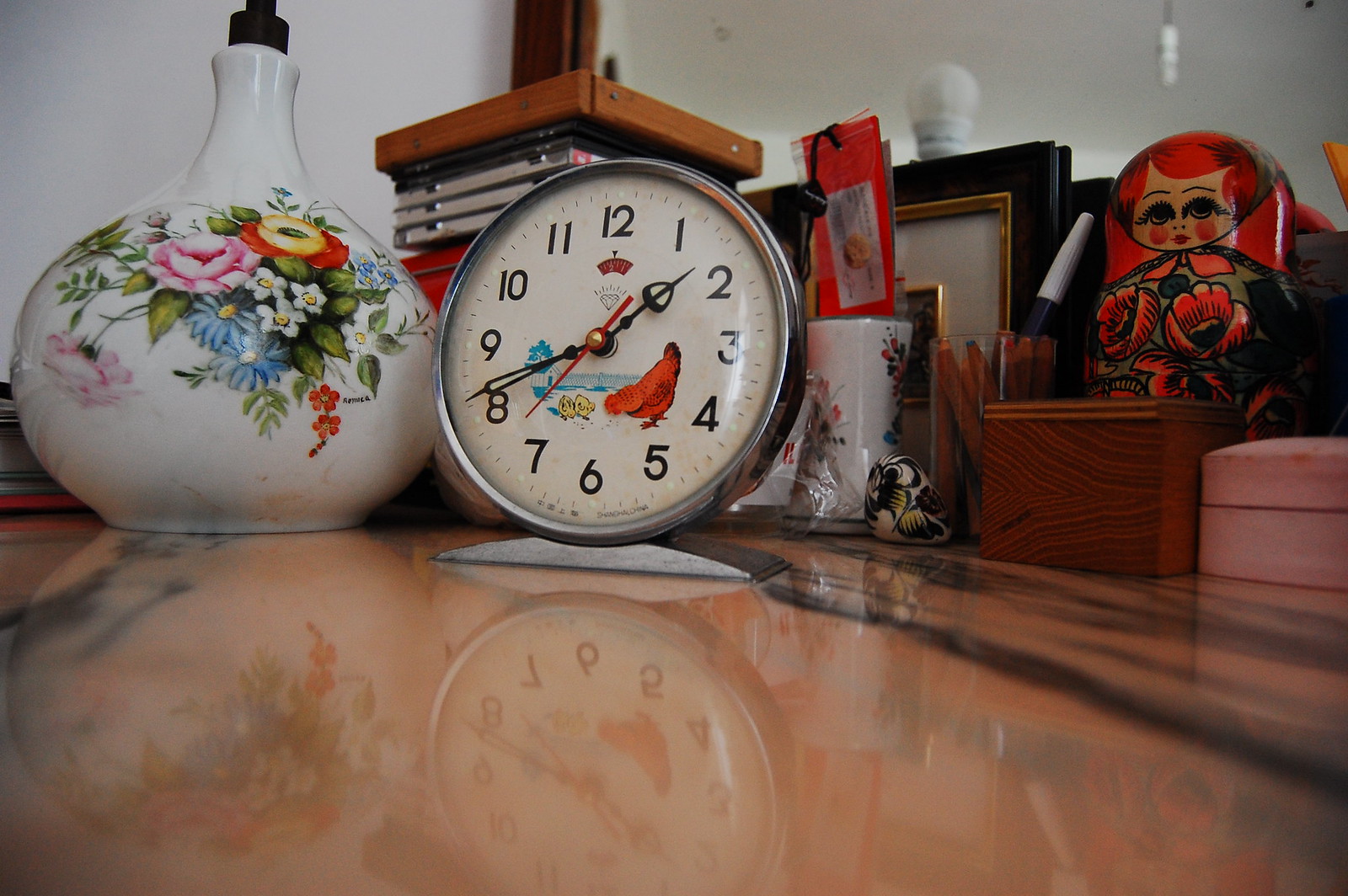The image is a high-resolution, landscape photograph depicting a collection of items placed on a highly reflective surface that resembles light brown marble with black veins. On the left side of the scene is an off-white flower vase filled with a mixed arrangement of flowers in pink, white, light blue, and red with yellow centers, surrounded by green foliage. Beside this vase is a silver-colored, round tabletop clock featuring an off-white face with standard black numerals (1 through 12), hour, minute, and second hands. The clock's center showcases an image of a red rooster standing beside a waterway. Behind the clock is a small CD tower with a wooden top, filled with several CDs. Toward the right, there is a picture frame with a plaque inside it. The polished stone surface beneath these objects creates clear reflections of each item.